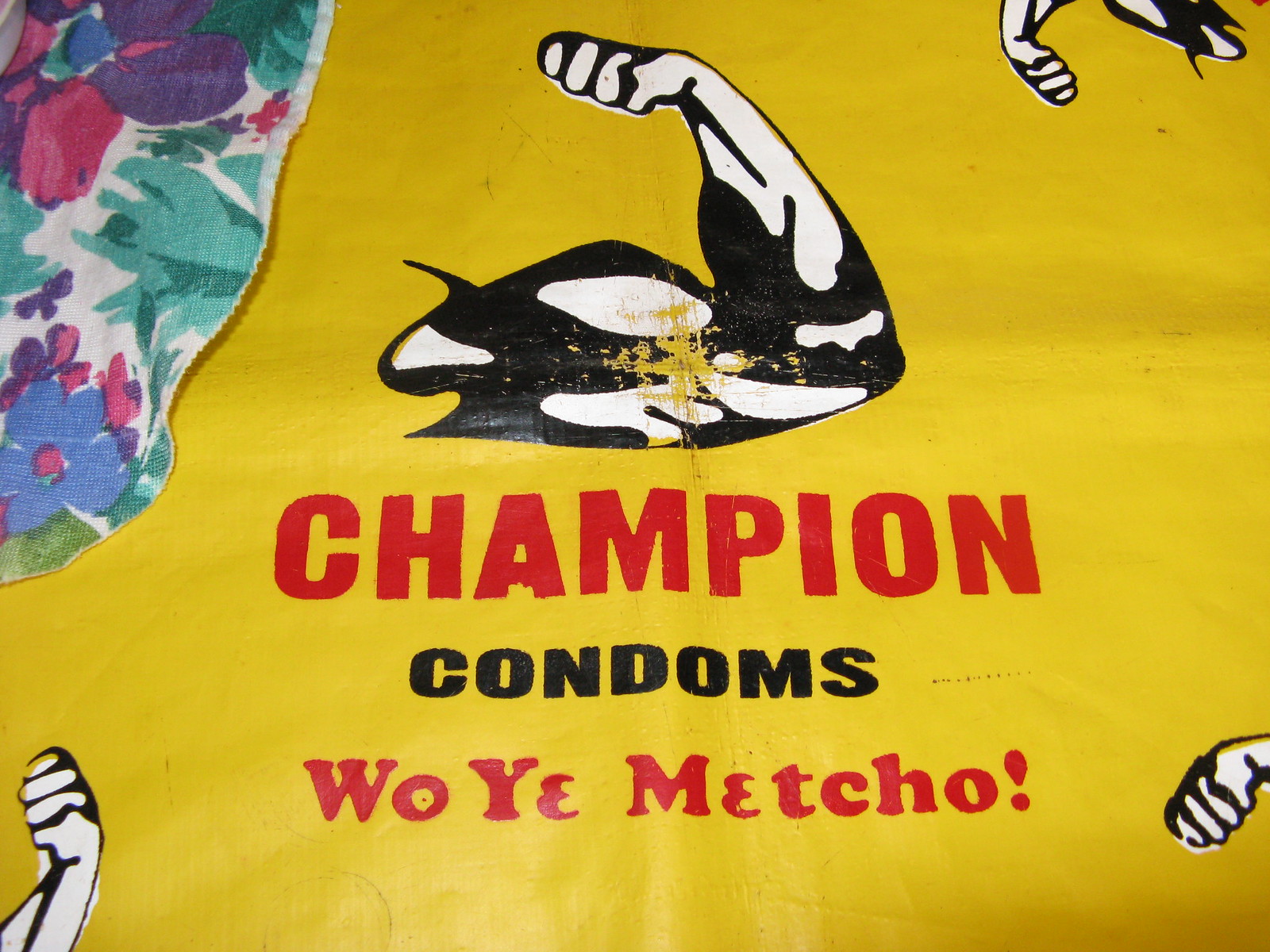The photograph features a vibrant yellow banner with striking details. Dominating the upper center is a cartoon illustration of a large, flexed bicep muscle, forming an L-shape and facing left. This muscular arm is black and features prominently in the design. In the upper left corner, a fabric patch adorned with red-purple flowers and green leaves is sewn onto the banner, adding a unique touch. Below the central bicep image, the banner displays text: the first line reads "Champion" in bold red letters, followed by "Condoms" in black text, and finally, "Bowie Metro!" in red text. The corners of the banner, excluding the upper left, feature partial images of flexed arms or fists, subtly extending the theme of strength and power across the composition.